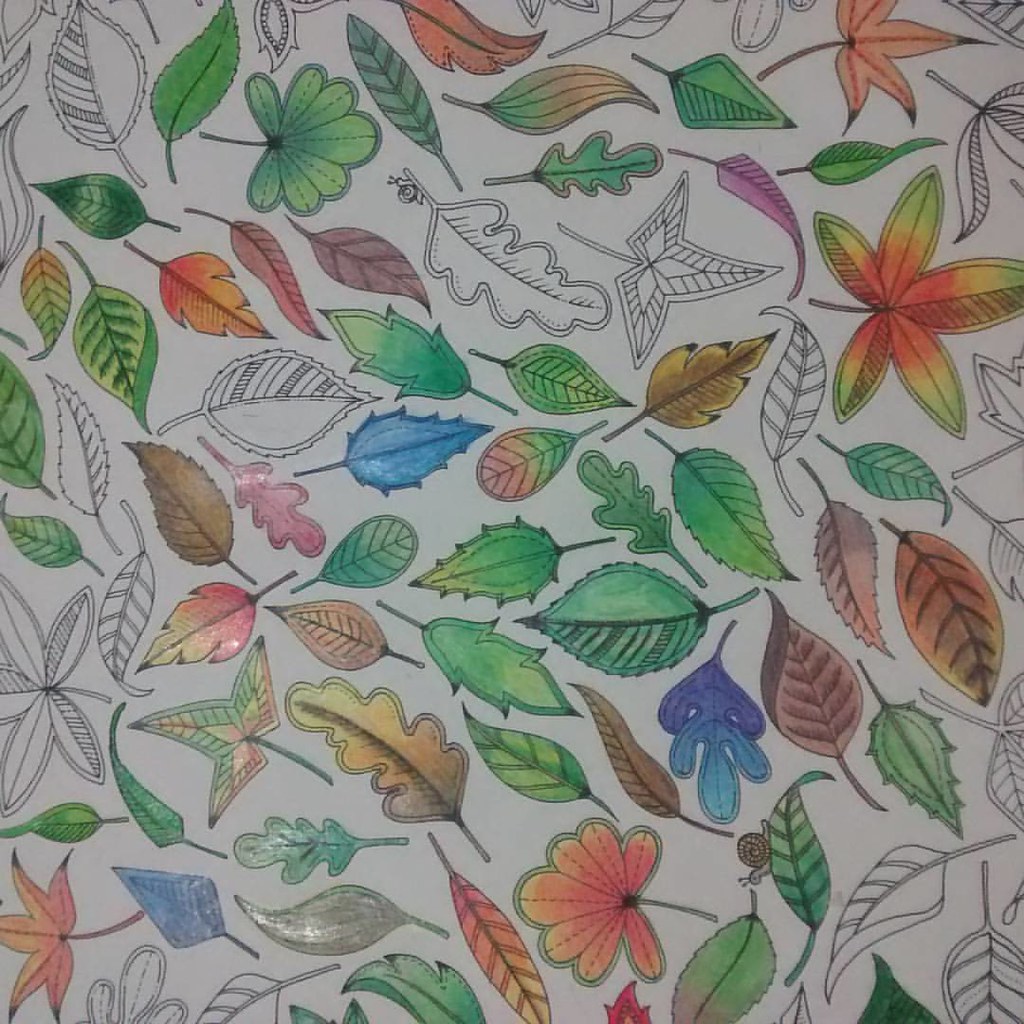The image showcases a close-up of a coloring book page filled with a diverse assortment of leaves, capturing the intricate and elaborate designs often found in adult coloring books. The leaves are depicted in a variety of types and are colored using an array of hues, including natural tones like various shades of green, autumnal oranges, reds, and yellows, as well as imaginative colors such as blues, purples, and teals. Some leaves remain uncolored, still in their black and white outlines, awaiting color. The leaves are scattered throughout the image, oriented in every direction—up, down, left, and right—covering the entire frame from corner to corner. A few small snails are also nestled among the leaves, adding whimsical detail. The overall scene is a vivid mosaic of color contrasted with areas of blank outlines, suggesting an ongoing creative process using crayons or markers.